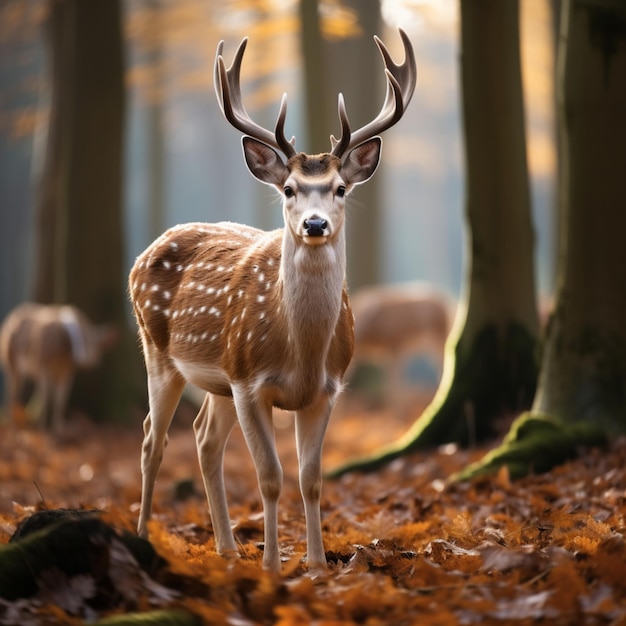This image appears to be a highly realistic drawing of a mature brown deer, possibly a four-point buck, which stands facing the viewer in a forest setting. The deer, with its characteristic light brown coat dotted with white spots, has a lighter underbody and neck, and a predominantly brown face with some white shading. It has large, black eyes, a black nose, and big floppy ears, with its head adorned by impressive brownish-gray antlers.

In the background, there are two more deer, slightly blurred but sharing the same coloration, suggesting depth in the scene. The ground is covered with reddish-orange leaves, indicating a fall setting, and the forest is dense with tall trees, some with moss growing on their trunks. The leaves on the ground resemble maple leaves, emphasizing the autumnal theme. Dim light filters through the trees, suggesting either early morning or late afternoon.